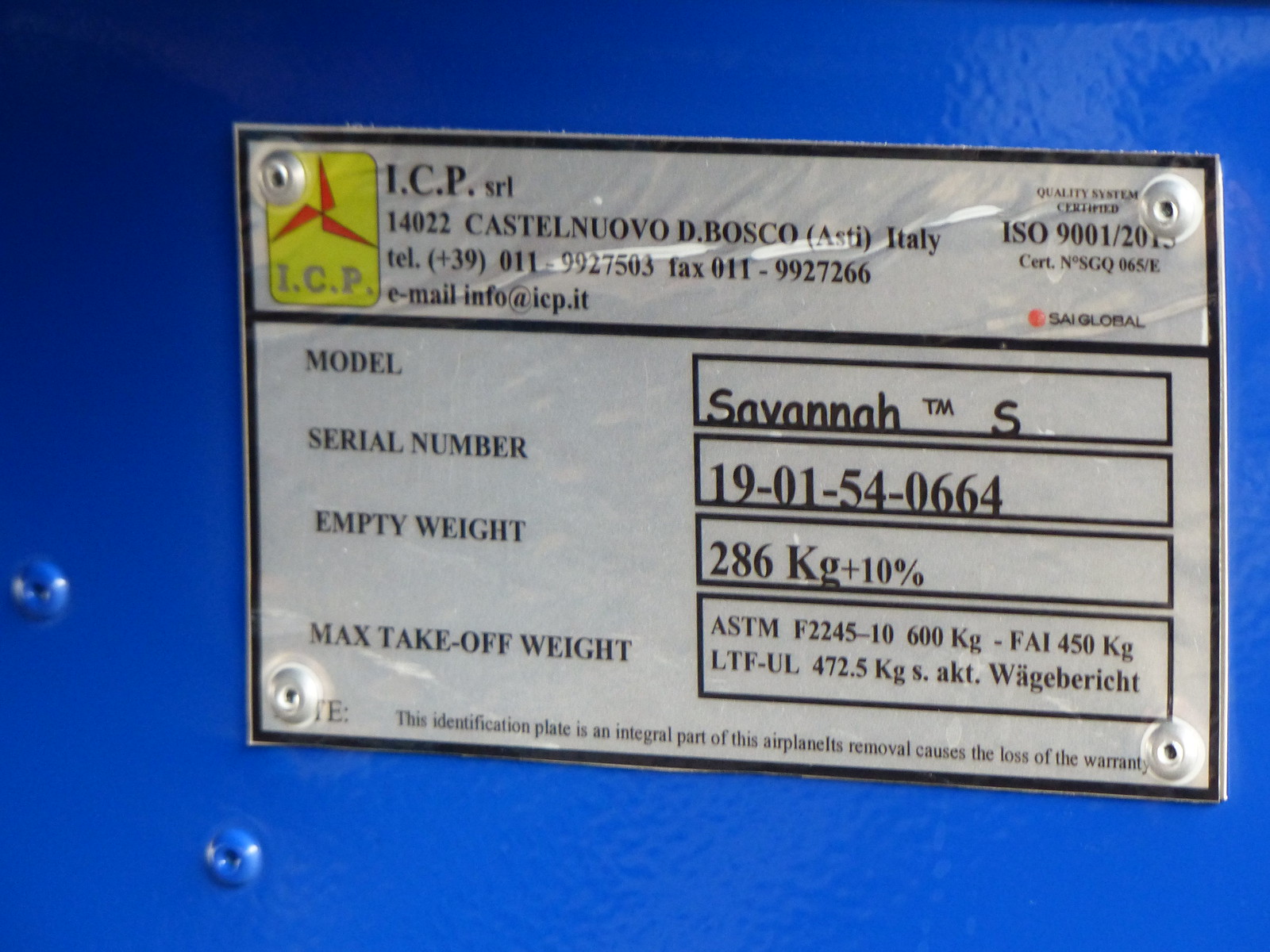This is a detailed close-up photograph of a manufacturing identification plate riveted onto a blue, powder-coated metal surface, likely part of an airplane. The silver metal plaque features a distinct black border and, in the upper right corner, a small yellow rectangle next to the black letters "ICP" and "ICP SRL 14022 Casalinova di Bosco, Asti, Italy." Below this are the company's telephone and fax numbers and their email address, info@icp.it, along with the certification "Quality system certified ISO 9001-2015."

On the left side of the plate, the information includes the airplane model, "Savannah TMS," with the serial number "1901540664." The empty weight is specified as "286 kg plus 10%," and the maximum takeoff weights are detailed as "ASTM 52245-10 600 kg," "FAI 450 kg," and "LTFUL 472.5 kg." Additionally, the plate bears a note that reads, "This identification plate is an integral part of the airplane. Its removal causes the loss of the warranty." This tag confirms that it is indeed associated with an airplane, providing vital specifications and contact information for the manufacturer.